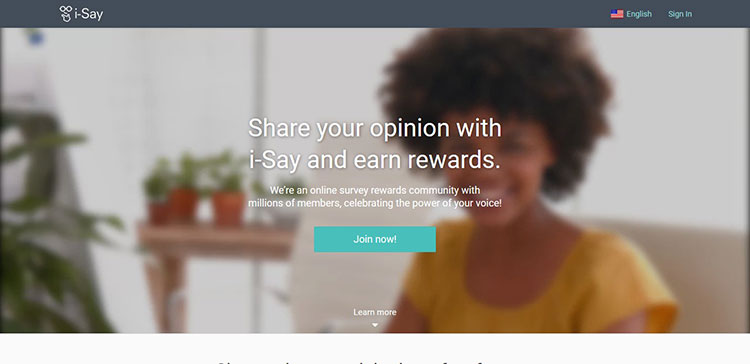A screenshot from a website features a header with a googly smiley face logo next to the text "i-say" in lowercase letters. In the upper right corner, there is an American flag icon followed by the word "English" and a "Sign in" link. The background is blurred to highlight the main content, which includes an African American woman with brown curly hair, smiling while wearing a short-sleeved yellow dress or shirt, standing in front of a shelf adorned with plants in orange pots.

Prominently displayed in white text, the image reads: "Share your opinion with i-Say and earn rewards." Below this in smaller print, it states: "We're an online survey rewards community with millions of members celebrating the power of your voice." There is a teal-colored button labeled "Join Now" and a "Learn More" link in white font at the bottom, accompanied by a downward-pointing arrow.